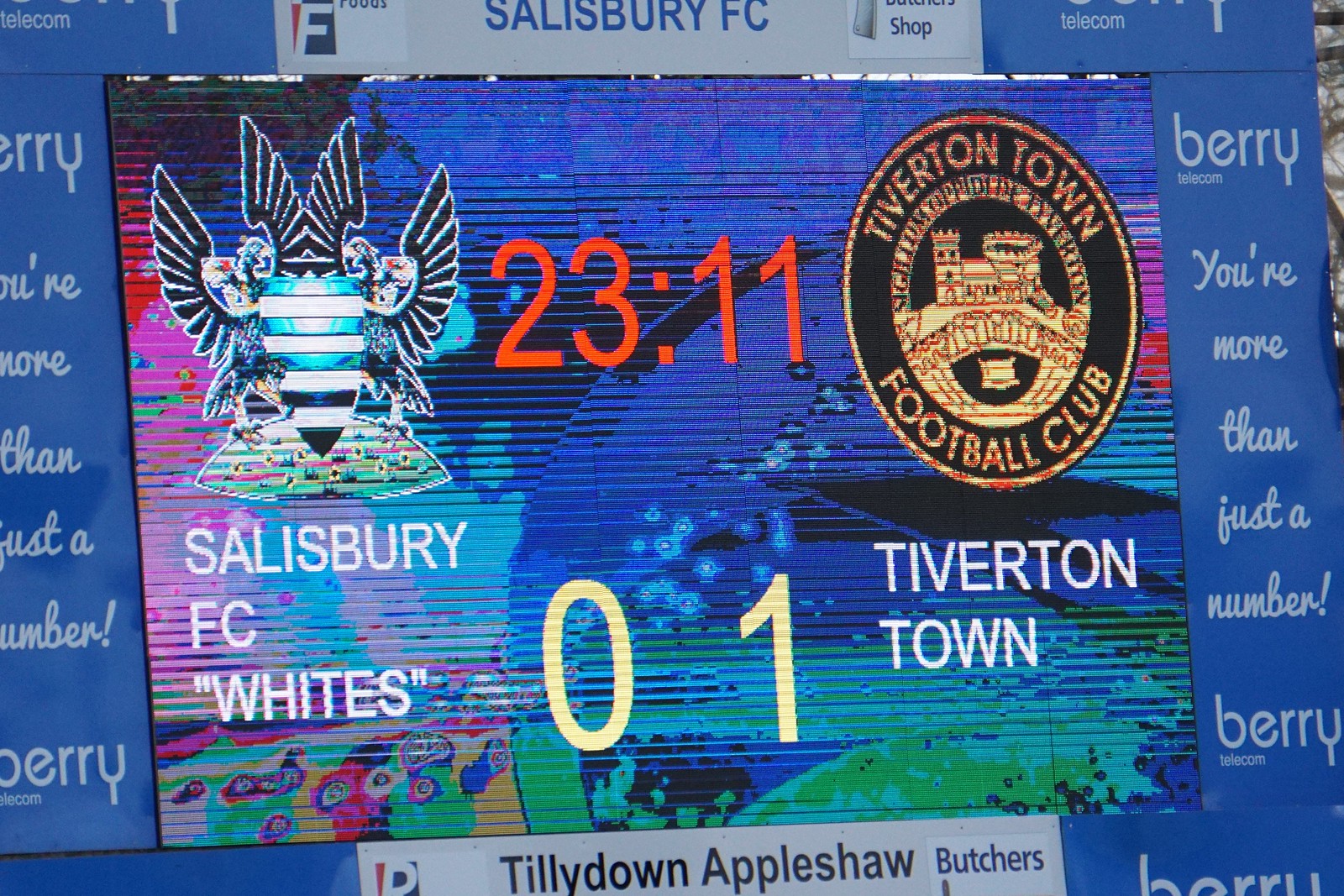The image shows a horizontally aligned rectangular scoreboard dominated by a blue background with numerous colorful accents, including purple, green, and orange, giving it a vibrant appearance. The top section features the name "Salisbury FC" in blue letters against a white strip. Below that, the left side of the scoreboard displays the emblem of Salisbury FC Whites, which resembles a winged trophy, while the right side showcases the emblem of Tiverton Town Football Club, depicting a black and gold castle.

Central to the scoreboard are large red numbers displaying “23:11,” indicating the time remaining in the match. Below this, it shows the current score with Salisbury FC at 0 and Tiverton Town at 1. Barry Telecom, presumably the sponsor, is prominently mentioned across the blue background with the slogan "Barry, you're more than just a number" repeated in white text. Additionally, a silver box below the main display advertises Tilly Down Appleshaw Butchers. The contrasting colors and various logos make the scoreboard both visually engaging and informative, giving a detailed overview of the ongoing soccer match between Salisbury FC and Tiverton Town.